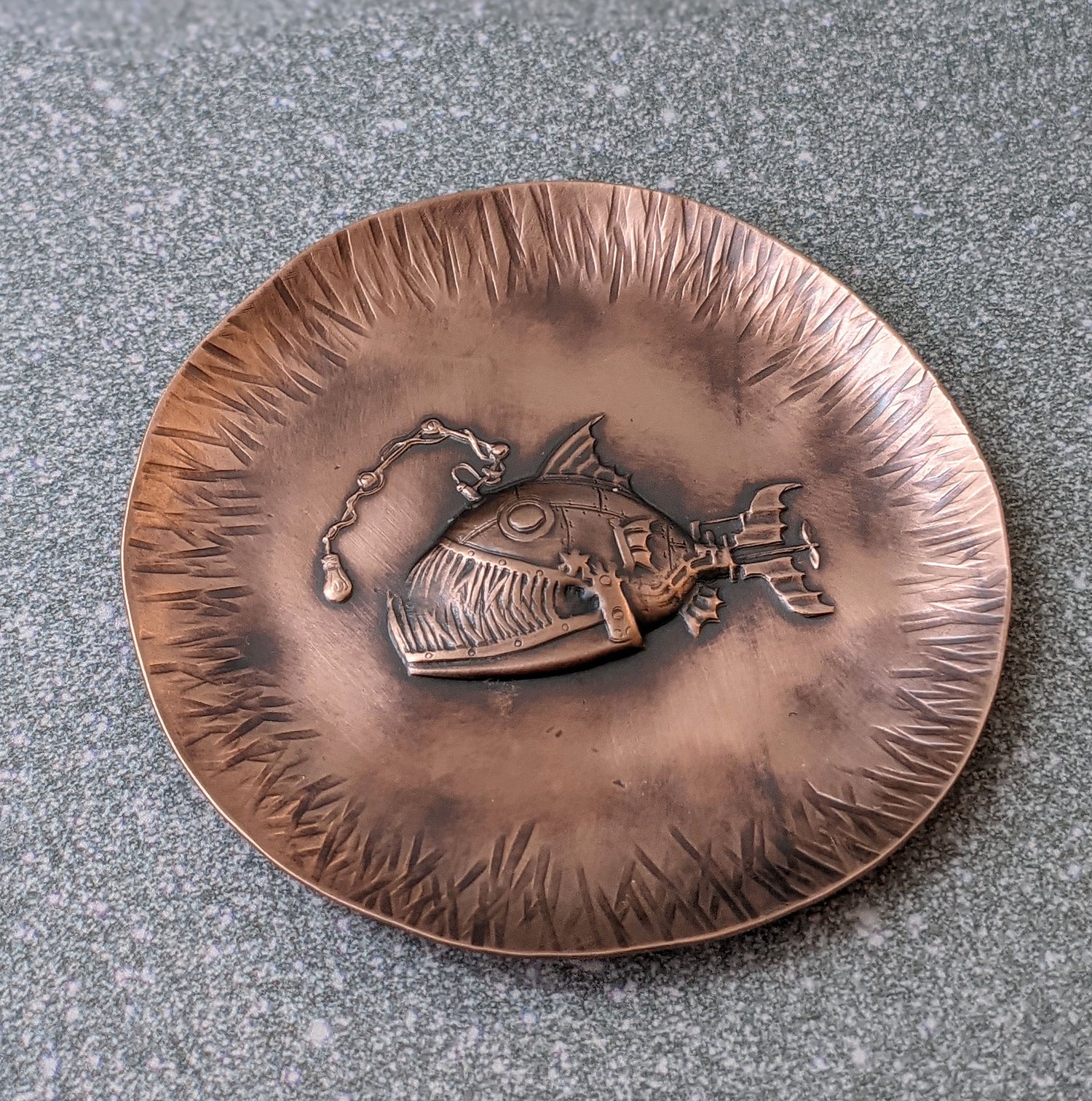The image showcases a captivating art piece, a copper plate placed on a gray and white speckled stone or granite table. The plate, with its bronze-ish hue and three-dimensional, tactile etching, features an intricately designed mechanical anglerfish as its centerpiece. This retro-punk styled anglerfish, crafted from metal, has various steampunk elements including a propeller tail fin, a hinged jaw with sharp teeth, and a light bulb substituting the traditional bioluminescent lure. The edges of the plate are lined with notched patterns, adding to the artistic decor. The mechanical anglerfish, complete with visible gears and mechanisms, appears almost as if piloted like a miniature ship, enhancing the surreal and imaginative quality of the piece.